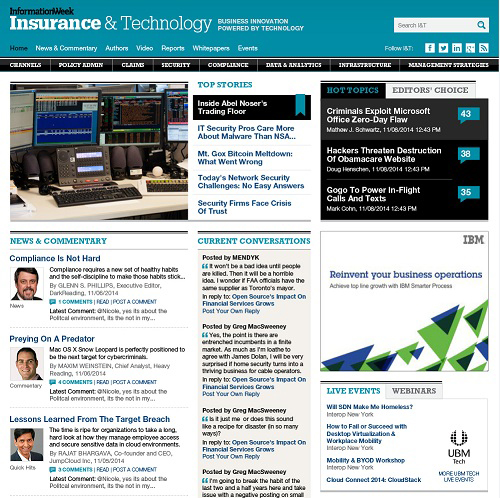This screenshot displays a webpage from a website titled "Information Week" located in the upper left-hand corner. The title is written in small black text, accompanied by a larger heading below that reads "Insurance and Technology." The word "Insurance" is highlighted in bold white text, while "Technology" is also in white but is followed by some unreadable text in white.

Positioned in the top right corner is a white search bar featuring a turquoise magnifying glass icon. Below the main title, categories are listed: "Home," "News and Community," "Authors," "Video Reports," "White Papers," and another word beginning with "Experts," which is unreadable.

On the upper right, a "Follow Us" section allows users to connect via social media platforms such as Facebook. Additional categories are listed horizontally across the page, though they are too small to decipher. An image of electronic devices, possibly two monitors and a laptop, is displayed, suggesting gaming purposes.

To the right of this image, a "Top Stories" section is displayed with four article titles listed vertically on a white background. Plus, a highlighted story features a headline on a black banner with a blue ribbon.

Further to the right, a black background section titled "Topics" includes three article titles, each accompanied by a blue chat box with numbers indicating comments or interactions. Another section labeled "Editor's Choice" follows underneath.

Beneath this, there are three men's photographs, with each providing news and commentary under a blue headline. The middle section, marked "Current Conversations," highlights popular discussion topics, and to the right, an IBM advertisement encourages users to "Reinvent Your Business Operations," with additional unreadable text.

At the bottom left, a series of blue and green arrows or triangular shapes overlap, leading downwards. The "Live Events" section lists upcoming webinars and events, while the "UBM" logo appears in the lower right corner, accompanied by unreadable text.